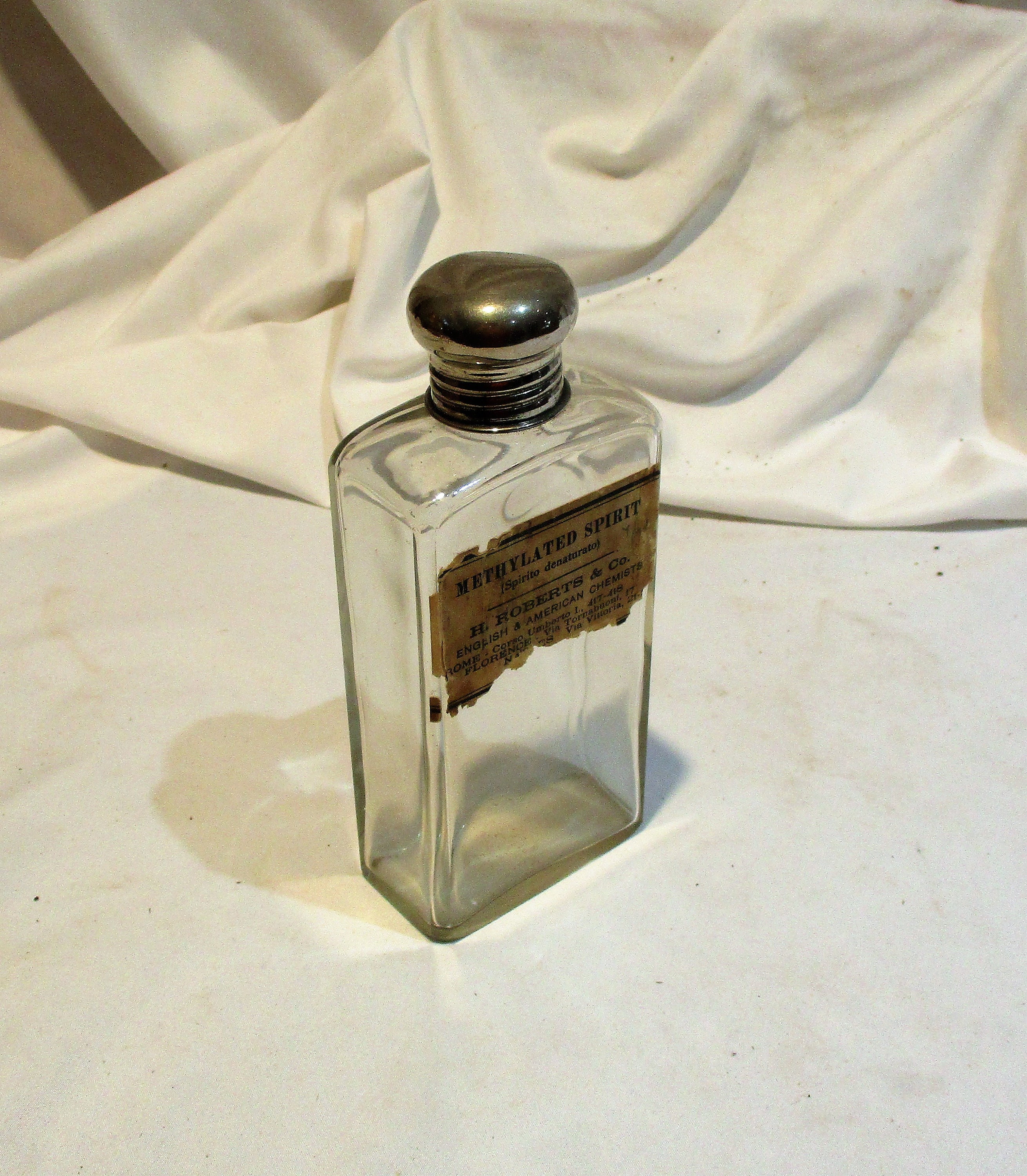The image displays an old, rectangular glass bottle with a rounded top, fitted with a shiny metal screw-on cap. The bottle, which is empty, rests on a piece of white fabric that appears stained and discolored. The fabric is taut at the bottom, with a more draped appearance in the background. The bottle’s vintage label, now faded and yellowed, is mostly peeled off but still partially legible, revealing the text “Methylated Spirit by H. Roberts and Co.” and additional words that are out of focus. The bottle casts a shadow on the fabric, further emphasizing its age and the overall worn look of the scene.